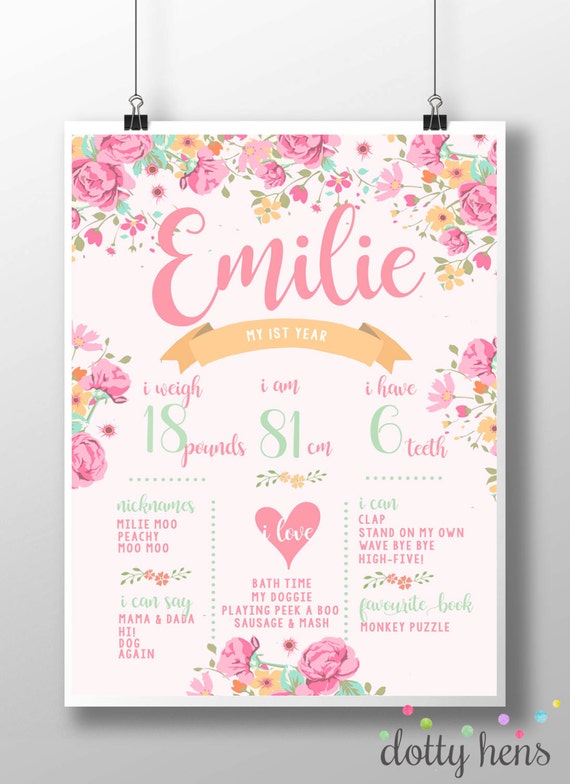This detailed infographic provides a comprehensive overview of a baby's first year. Suspended from black binder clips against a light gray wall, the white paper is elegantly bordered with pink, blue, yellow, and orange flowers. At the top, "Emily" is written in large pink cursive, followed by a light orange banner that states "My First Year." Three key facts are highlighted: "I weigh 18 pounds," "I am 81 centimeters," and "I have six teeth," with the numbers prominently in green.

Below these facts are sections separated by small dots and detailing various aspects of Emily's life. Her nicknames include "Millie Moo," "Peachy," and "Moo Moo." She can say "mama," "dada," "hi," "dog," and "again." Emily loves bath time, her doggie, playing peek-a-boo, and eating sausage and mash. Her abilities include clapping, standing on her own, waving bye-bye, and giving high-fives. Her favorite book is "Monkey Puzzle." The bottom right corner of the infographic bears the name "Dottie Hens."